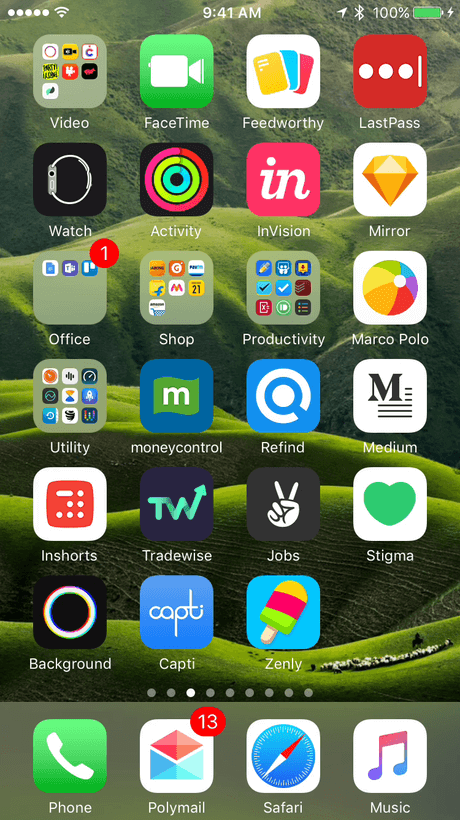This image features a vibrant green background depicting expansive rolling hills with several small buildings nestled at the bottom. At the top of the image, there are five small white circles. The device's status bar indicates the time as 9:41 a.m., a fully charged battery at 100%, and a strong signal. The home screen is filled with numerous app icons, including Video, FaceTime, Feedworthy, LastPass, Watch, Activity, Envision, Mirror, Office (marked with a red notification circle containing the number 1), Shop, Productivity, Marco Polo, Utility, Money Control, Refined, Medium, In Shorts, TradeWise, Jobs, Stigma, Background, Capti, and Zenly. Additionally, there are white dots across the bottom indicating multiple app pages, with the third dot lit white. At the bottom of the screen is a large gray box housing the Phone app, Polymail (displaying a red notification circle with the number 13), Safari, and Music.